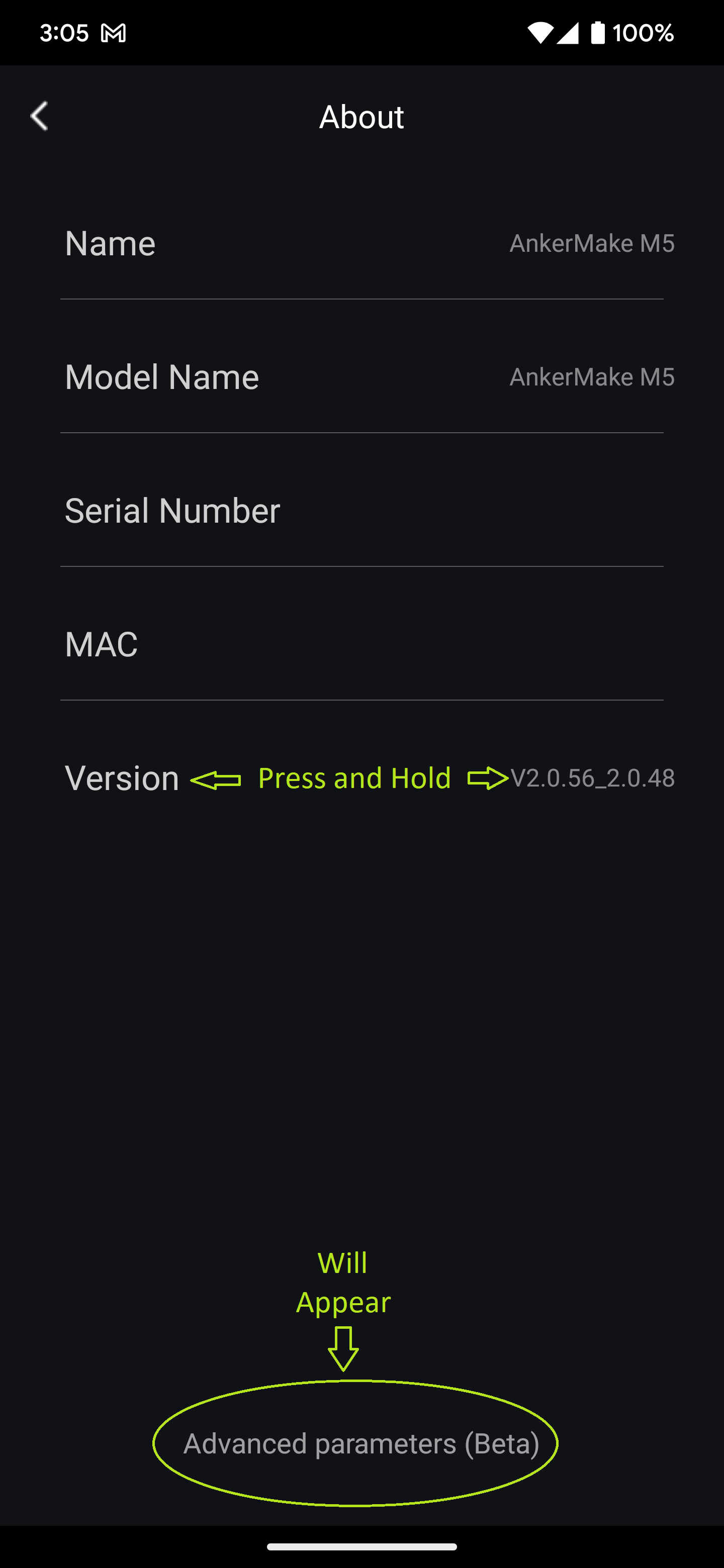This detailed screenshot captures the display from a phone's screen with a predominantly black, vertical rectangle interface. In the upper left corner, the white text indicates the time "3:05." To the upper right, icons symbolize the internet connection and a fully charged battery at 100%.

Central to the image, the text "Model Name: Ankermake M5" appears twice - once under a heading, and again with smaller details following it. Beside the model name, the text includes "Serial Number" and "MAC" followed by specific information not shown in the description. 

Below these details, the word "Version" is highlighted, emphasized by a green arrow pointing toward it from the right. A directive, "Press and Hold," appears with an accompanying arrow pointing to the right and another pointing to the left, suggesting actionable elements.

Near the bottom of the interface, a phrase "Advanced Parameters (Beta)" is encircled by a large, green oval. Just above this oval, the words "Will Appear" are displayed, with a downward arrow pointing directly at the encircled phrase, indicating that additional options might be revealed upon selection.

This thorough description provides a clear representation of the on-screen elements captured in this phone screenshot.